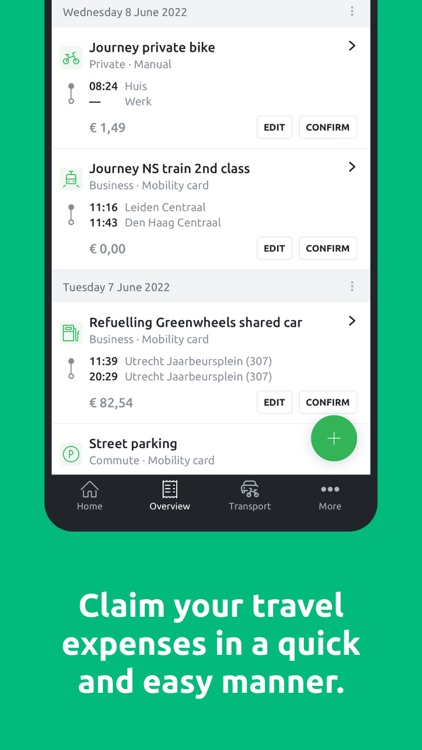In this image, an advertisement centered around a mobile phone screenshot is displayed. At the top of the screenshot, the date "Wednesday, 8th June 2022" is prominently featured. Below this, the text reads, "Journey private bike for 149 euros." Next, it states, "Journey NS train second class business mobility card" alongside a cost of "0 euros." 

Following this, another date, "Tuesday, 7th June 2022," is shown, accompanied by the expense "Refueling green wheels, shared car, 82.54 euros." At the bottom of the screenshot, it mentions "street parking." Just above the phone's screen, there is a green circle with a plus sign symbol situated near the bottom right.

Along the bottom edge of the phone's screen, there are four buttons labeled: "Home," "Overview," "Transport," and "More." Beneath the phone screen, white text on a green background states, "Claim your travel expenses in a quick and easy manner." The green background color extends upward, forming a frame around the phone.